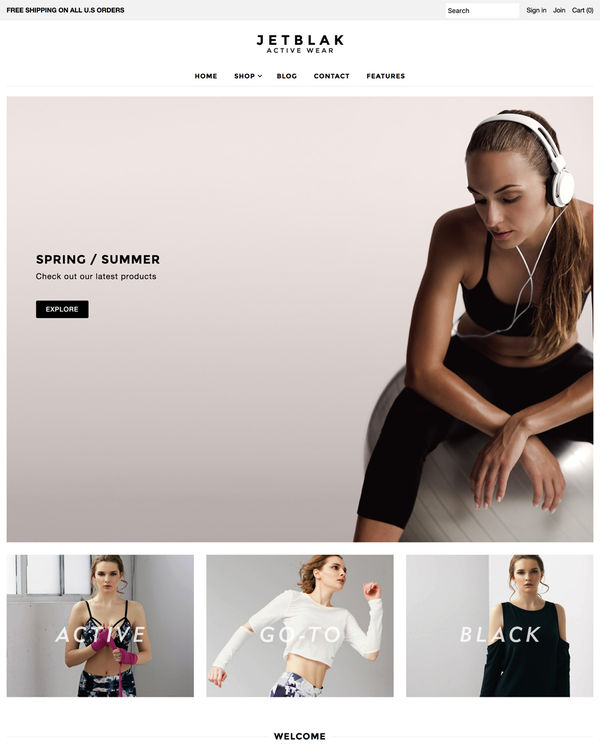Screenshot of an e-commerce website featuring fitness and activewear. The webpage has a clean, white background. At the top of the page, there is a navigation menu with the options: "Black and Active Wear," "Home," "Shop," "Blog," "Contact," and "Features." A large banner announces "Free Shipping on all US orders" and includes a search bar for easy navigation. Users can also find "Sign In" and "Join" links, along with a shopping cart icon displaying a zero, indicating no items in the cart.

Below the navigation menu, on the left side, a beige square highlights the text "Spring/Summer: Check out our latest products." Adjacent to it, a prominent black rectangle contains the inviting phrase "Explore in White." The main image features a woman comfortably seated on a grey exercise ball. She wears headphones, reinforcing the activewear and fitness theme.

At the bottom of the screenshot, there are three smaller images that serve as links to various sections, labeled "Active," "Go To," and "Black." Additionally, a footer showcases the word "Welcome" in black, visually tying together the overall professional and sleek design of the webpage.